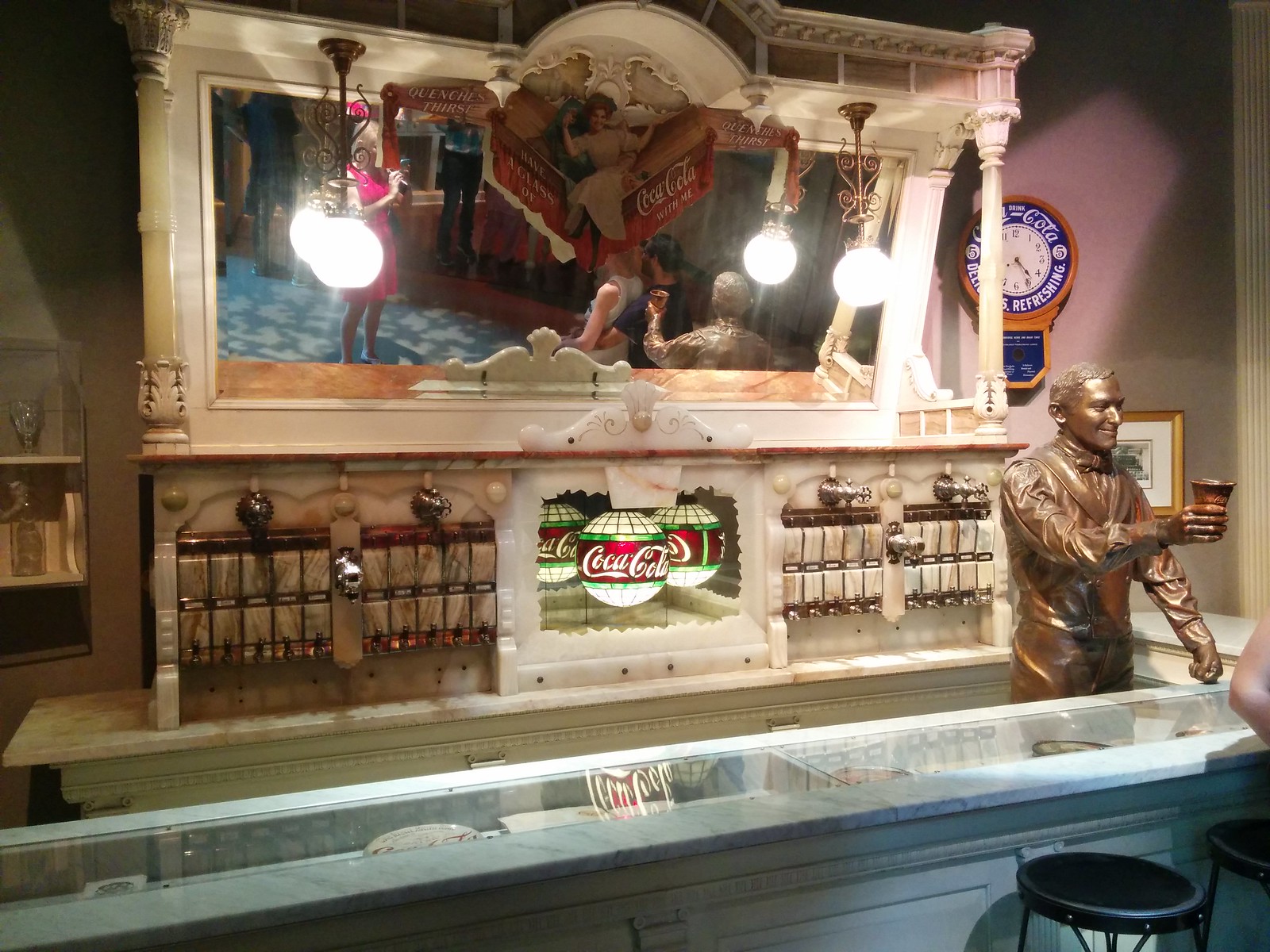The image depicts an elaborate, decorative bar, potentially located in a theme destination or museum setting, featuring an array of intricate details that showcase a Coca-Cola motif. The bar itself is tall and made predominantly of marble, with a glass case integrated into its top, framed by light blue cabinetry. On both the left and right sides of the bar are round pendant lights, and scattered throughout are various Coca-Cola decorations including globes and a notable clock on the right purple wall that reads around 4:25.

Central to the scene is a large, ornate mirror tilted downward, reflecting several figures. A woman in a pink dress holds a microphone, suggesting she is conducting an interview, while another woman in a pink dress appears to be taking a picture. Nearby, a man in a red and black shirt poses. Below this mirror are numerous spigots—four on each side with 20 different flavor options, and an additional spigot centered beneath the Coca-Cola emblem.

Adding to the eclectic mix is a bronze statue dressed in an old-style tuxedo, holding up a glass of Coca-Cola with a smile. Positioned behind the marble bar, the statue stands out as a prominent feature. The bar's decorative elements—including small gold frames and black stools—combine to create a vibrant, nostalgic atmosphere that underscores its likely theme-focused or commemorative nature.